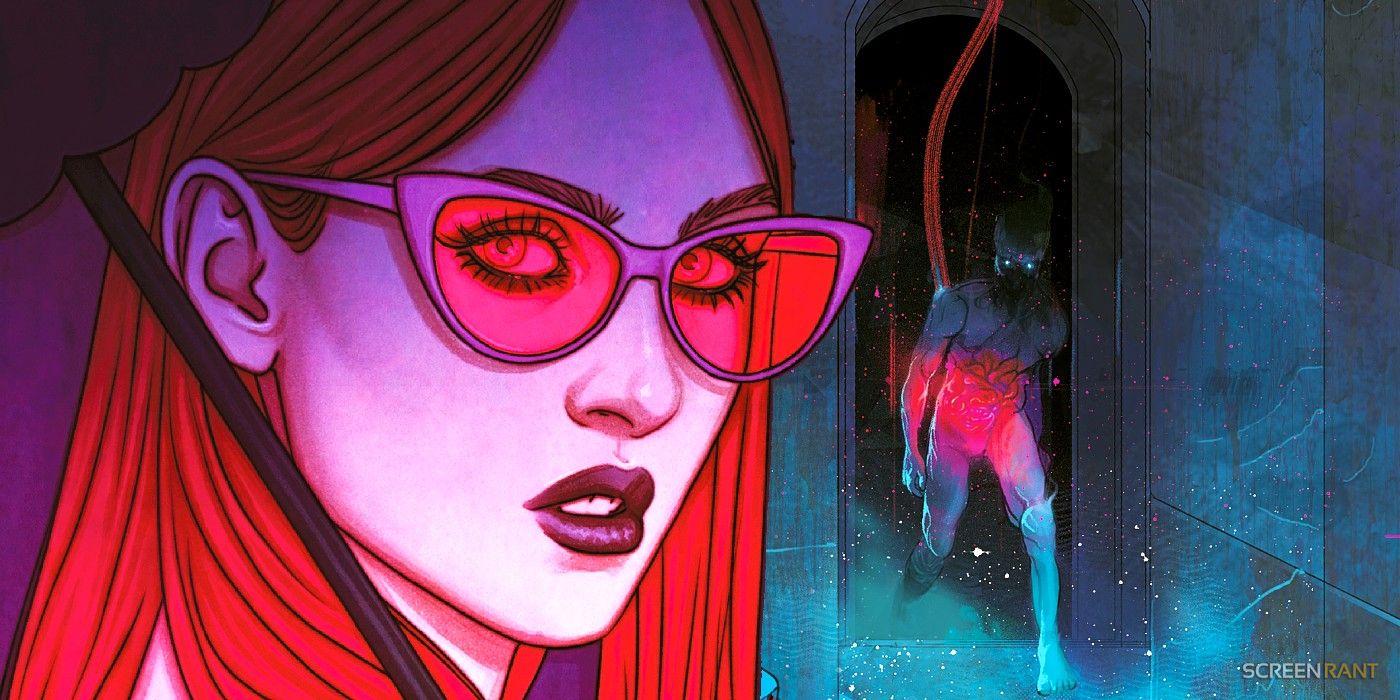This digital illustration, reminiscent of a science fiction cartoon, is presented in a narrow, wide landscape orientation. On the left side of the image, a young woman with long, orange hair cascading past her shoulders is depicted with a close-up view from her forehead to just below her chin. She gazes upwards with her mouth slightly open, her head turned back toward the viewer. She sports lavender cat-eye glasses with dark orange lenses, casting an orange hue over her eyes. Her eyelashes or eyebrows are accentuated with mascara, giving them an elongated appearance. A stick or umbrella is slung over her left shoulder, the top peeking out at the upper left of the image.

On the right side, a sinister, devil-like creature is emerging from a dark, arched hallway. The creature appears to be a hybrid, featuring both human and dog-like characteristics. Its red glowing tail arches over its back, and its stomach exudes a red glow. The creature’s beady, white-lit eyes fixate on the viewer menacingly. It is clad in tall white boots but otherwise appears unclothed. The background features a blue-toned stone wall, and the bottom right corner of the image bears the text "screen rant" in gold lettering. The entire scene is vividly colored, adding to its surreal and otherworldly atmosphere.